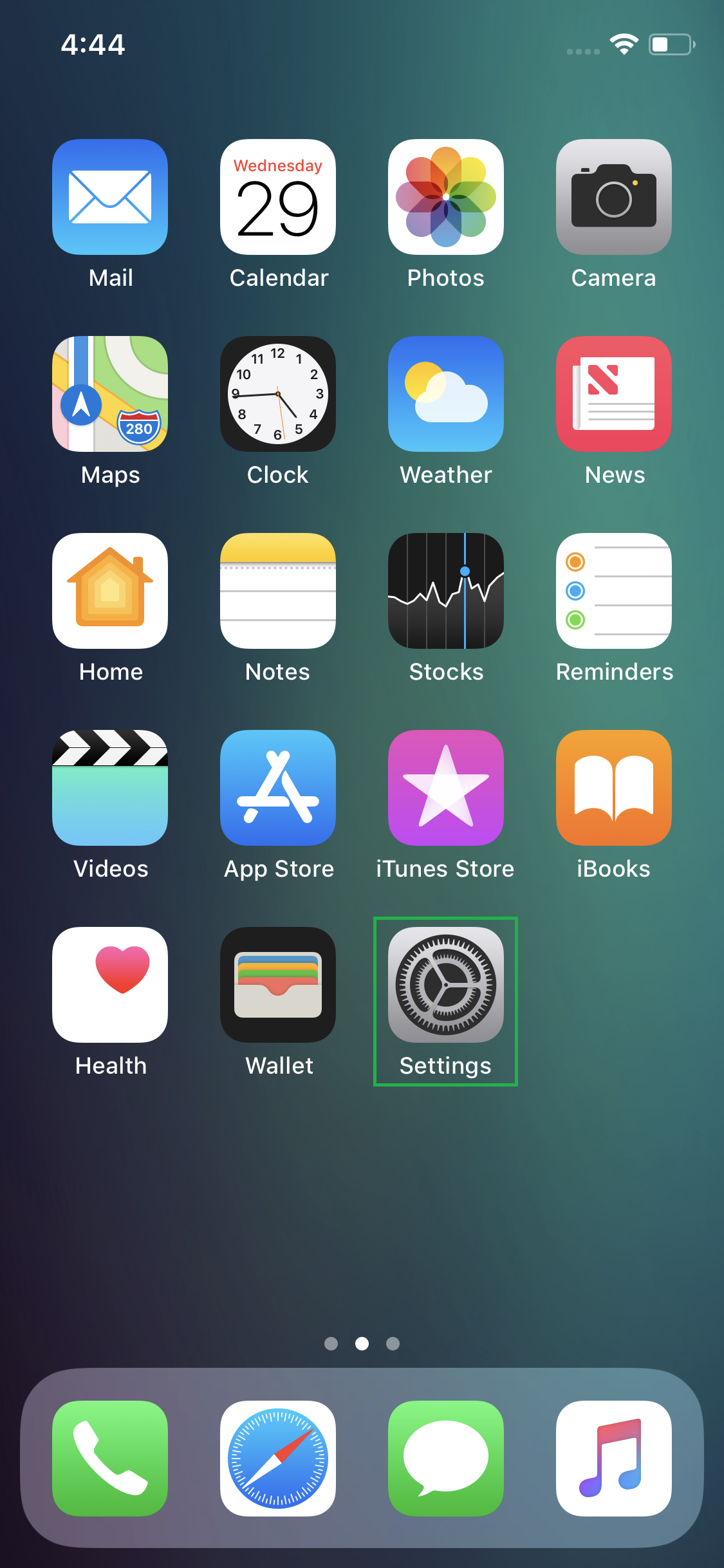In the image, the background is artistically divided with a gradient, transitioning from gray on the right to black on the left, creating a visually appealing blend. The focal point of the image is a smartphone displaying a screenshot. Occupying the top left corner of the screen is the number "4:44," indicating the time, while the top right corner features an ellipsis menu alongside indicators for Wi-Fi connectivity and a battery level at approximately 50%.

Immediately below these indicators, the main interface of the smartphone reveals an array of app icons neatly organized in rows of four. Each icon is housed within a square, accompanied by a descriptive label underneath. The first row of icons includes: "Mail," "Calendar," "Photos," and "Camera." Following that, the second row comprises: "Maps," "Clock," "Weather," and "News." The third row displays: "Home," "Notes," "Stocks," and "Reminders." In the fourth row, the icons are: "Video," "App Store," "iTunes Store," and "Books." Lastly, the fifth row presents: "Health," "Wallet," and "Settings," with one blank space remaining.

At the very bottom of the screen, three horizontal dots are centrally aligned, suggesting a paginated interface with additional screens. Just below these dots, there's a dark gray, oblong area featuring four more icons arranged side by side. This setup provides a comprehensive and orderly view of the smartphone's interface against the contrasting backdrop.